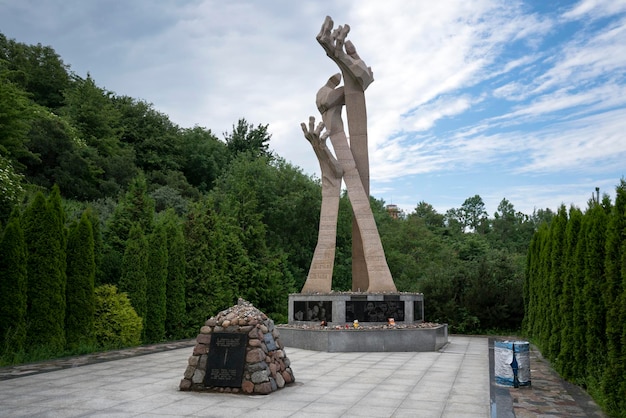The photograph captures a vibrant outdoor plaza surrounded by lush, dense trees under a partly cloudy, blue sky. The central focus of the image is a large, abstract stone sculpture featuring three outstretched, tan-colored hands that twist around each other as they reach skyward. The hands ascend from a cement base, adding to the statue’s imposing height. In front of this unique art piece, there is a carefully arranged mound of stones and a plaque with text, though the details of the writing remain unreadable in the image. This stone mound may contain additional interpretive information about the artwork. The plaza itself is paved with flat stones, creating a spacious patio area amid what appears to be a woodland setting. A slight hill can be observed on the left side of the image, rising out of the frame. The overall scene captures a blend of natural beauty and intriguing, possibly enigmatic, artistry.